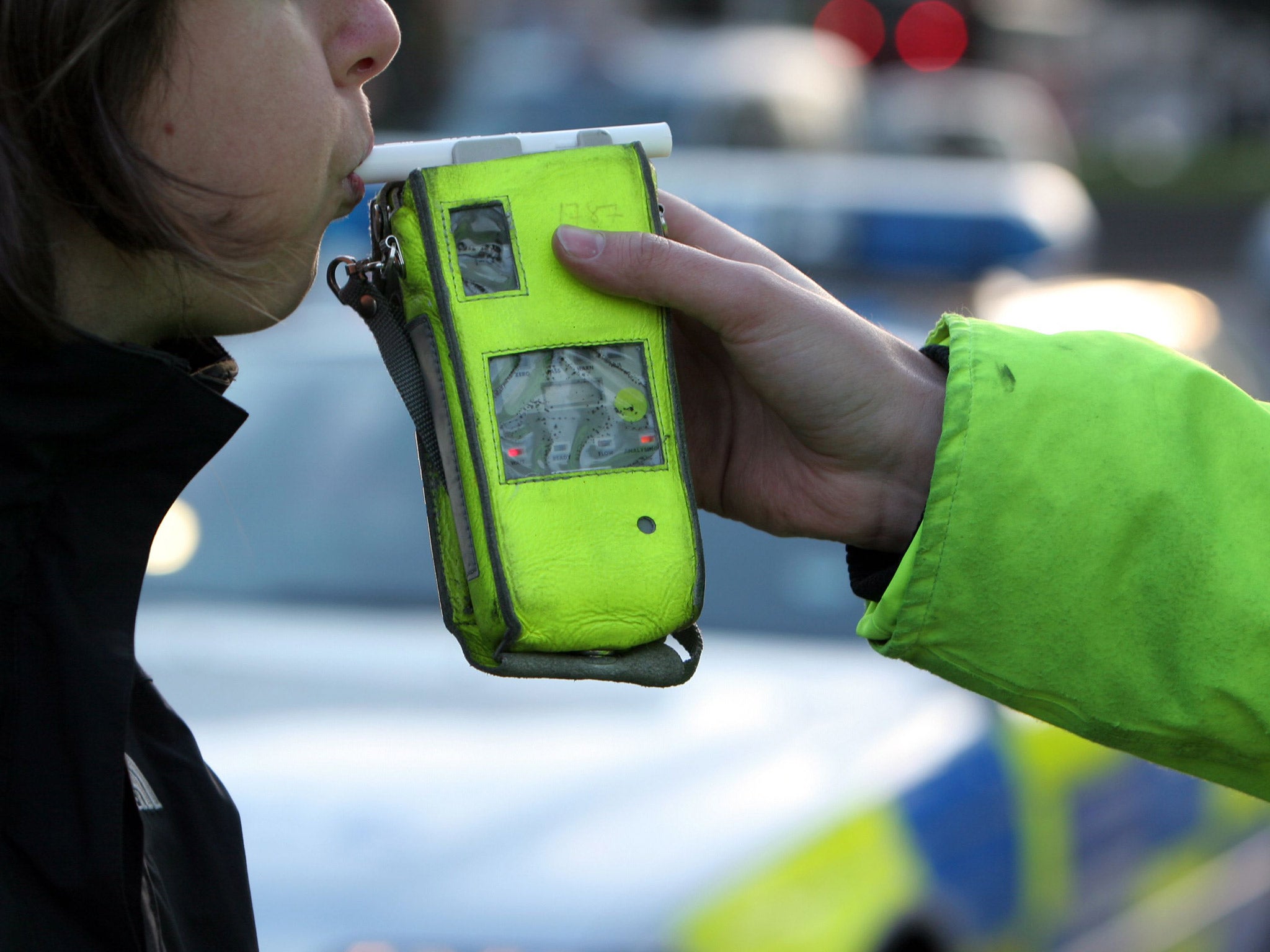A person is depicted in the act of taking a breathalyzer test. The focal point of the image is a brightly colored breathalyzer device, held by an outstretched arm clad in a neon green or yellow jacket sleeve. The hand gripping the device is bare. The breathalyzer itself is rectangular, vertically oriented, and vivid yellow, featuring a black strap on its side and a white tip that resembles a cigarette. The individual taking the test is partially visible, with only the lower half of their face showing, revealing short dark brown hair and a black jacket. In the blurred background, a police car can be faintly seen, predominantly white with yellow and blue markings on its side, and equipped with horizontal lights on its roof.